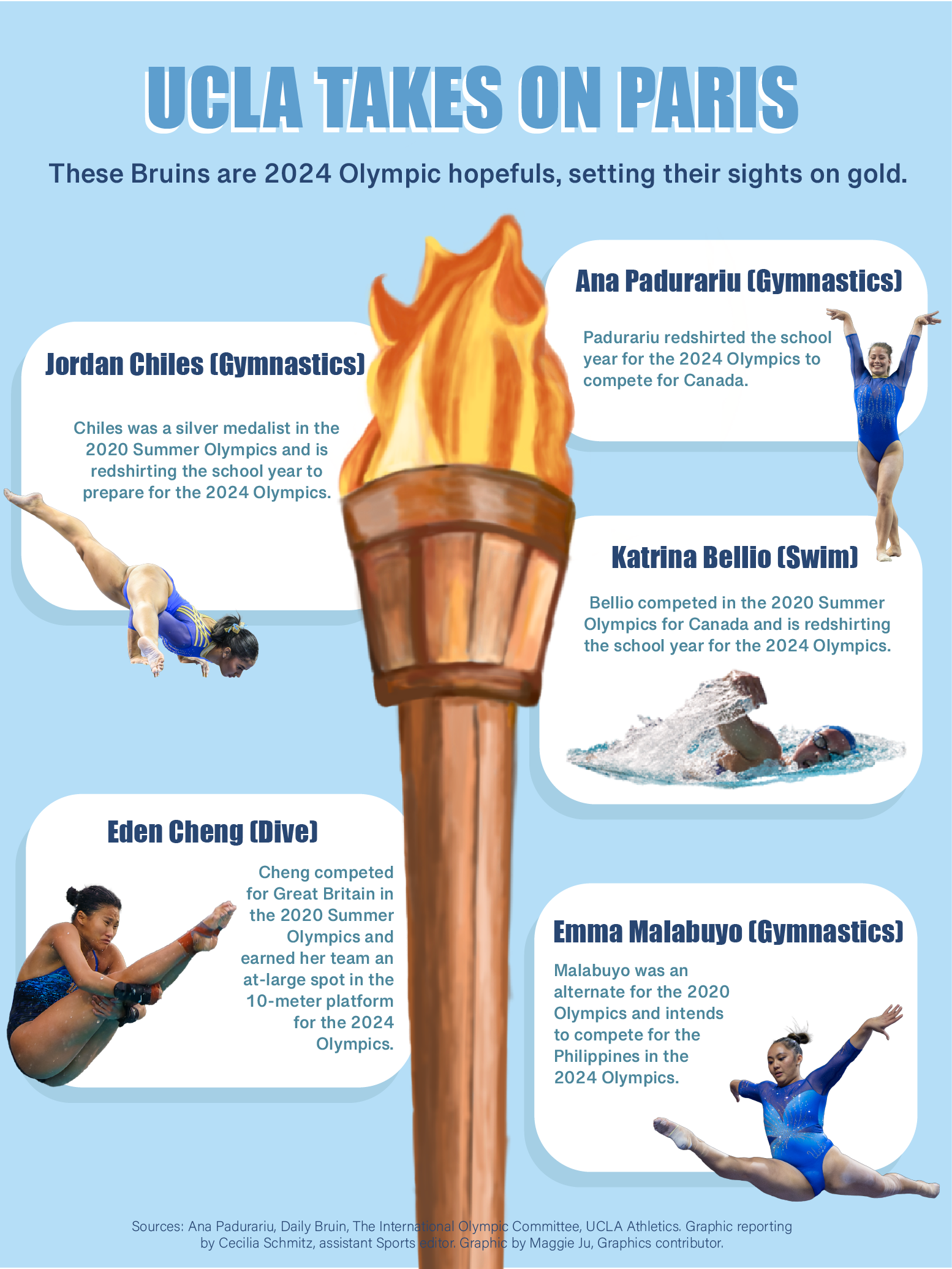The advertisement poster features a light blue background with the bold headline "UCLA Takes on Paris" at the top in a slightly darker blue. Below it, the subheading reads, “These Bruins are 2024 Olympic hopefuls, setting their sights on gold.” Dominating the center of the poster is an illustrated Olympic torch, stretching from near the bottom to just below the headline. The poster spotlights five UCLA athletes, each pictured in action within white boxed frames:

- On the left, Jordan Childs, a gymnast, is positioned above Eden Chang, a diver competing in the Dive Olympics.
- On the right, Ana Padurario, another gymnast, is shown above Katrina Bellow, a swimmer competing in the swimming competition.
- Beneath them, Emma Malabuyo is featured in her gymnastics discipline.

Each athlete’s name is accompanied by a single line of text detailing their sport. At the bottom of the poster, there is smaller print for additional information. The design exudes a sense of ambition and pride as these athletes aim for gold in the 2024 Olympics.